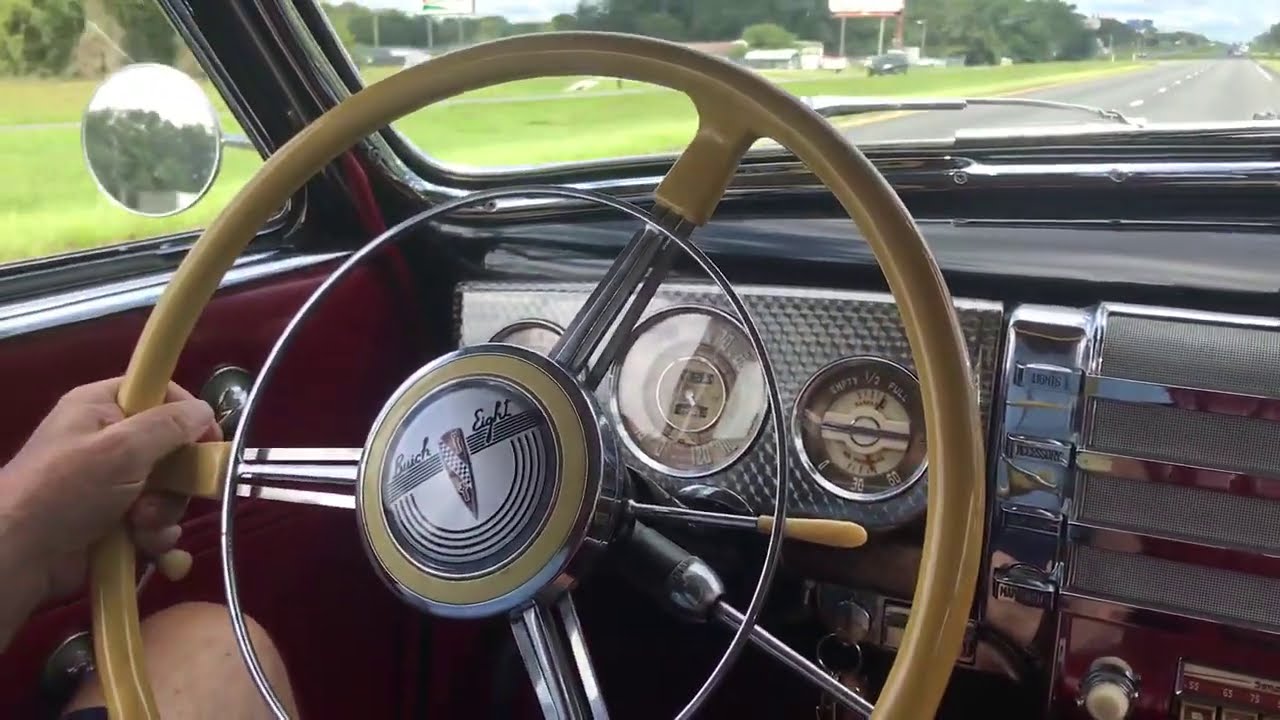This photograph depicts the interior of a restored vintage car, identified as possibly a Buick Super. Dominating the scene is a distinctive steering wheel, which features a yellow, mustard-colored outer ring and chrome metal arms extending to the wheel's center. The center of the steering wheel showcases the classic Buick 8 logo and text, flanked by gold and chrome rings. A hand grips the wheel, guiding the car down a clear road. The driver's side door panel is a rich red leather, adding to the nostalgic feel.

Ahead of the wheel are vintage dials and meters, set against what seems to be a carbon fiber-look dashboard, providing an elegant contrast in appearance. Chrome knobs and a vintage radio highlight the meticulous restoration of this classic interior.

Looking through the car's window, the road is visible, bordered by grassy areas and a line of trees in the distance. Small buildings are scattered further back, framed by a blue sky, adding a serene backdrop to this nostalgic driving experience.